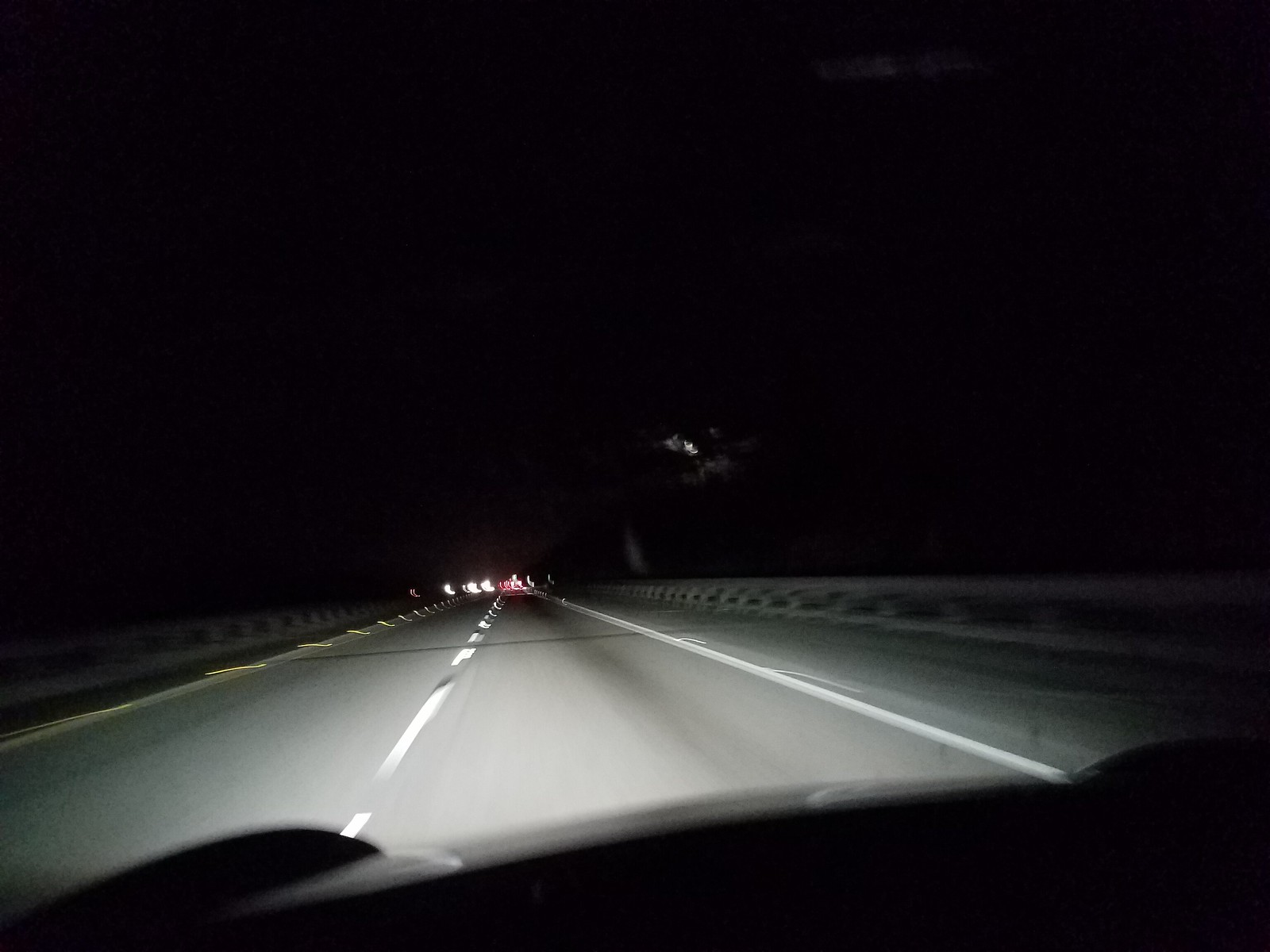This nighttime photograph captures the view from inside a moving vehicle, looking out through the windshield. The dashboard is partially visible at the bottom of the image, subtly illuminated by the car's interior lights. The road ahead, a two-lane highway, is faintly lit by the vehicle's headlights. Guardrails line both sides of the road, and the white painted dotted line in the center separates the lanes, while a solid white line marks the right shoulder. In the distance, blurred red and yellow lights hint at other vehicles, and faint oncoming white headlights can be seen. The moon peeks through darkened trees along the roadside, casting a gentle, diffused glow over the scene. The overall image is largely cloaked in darkness, accentuated by the limited light sources from the car and distant vehicles.